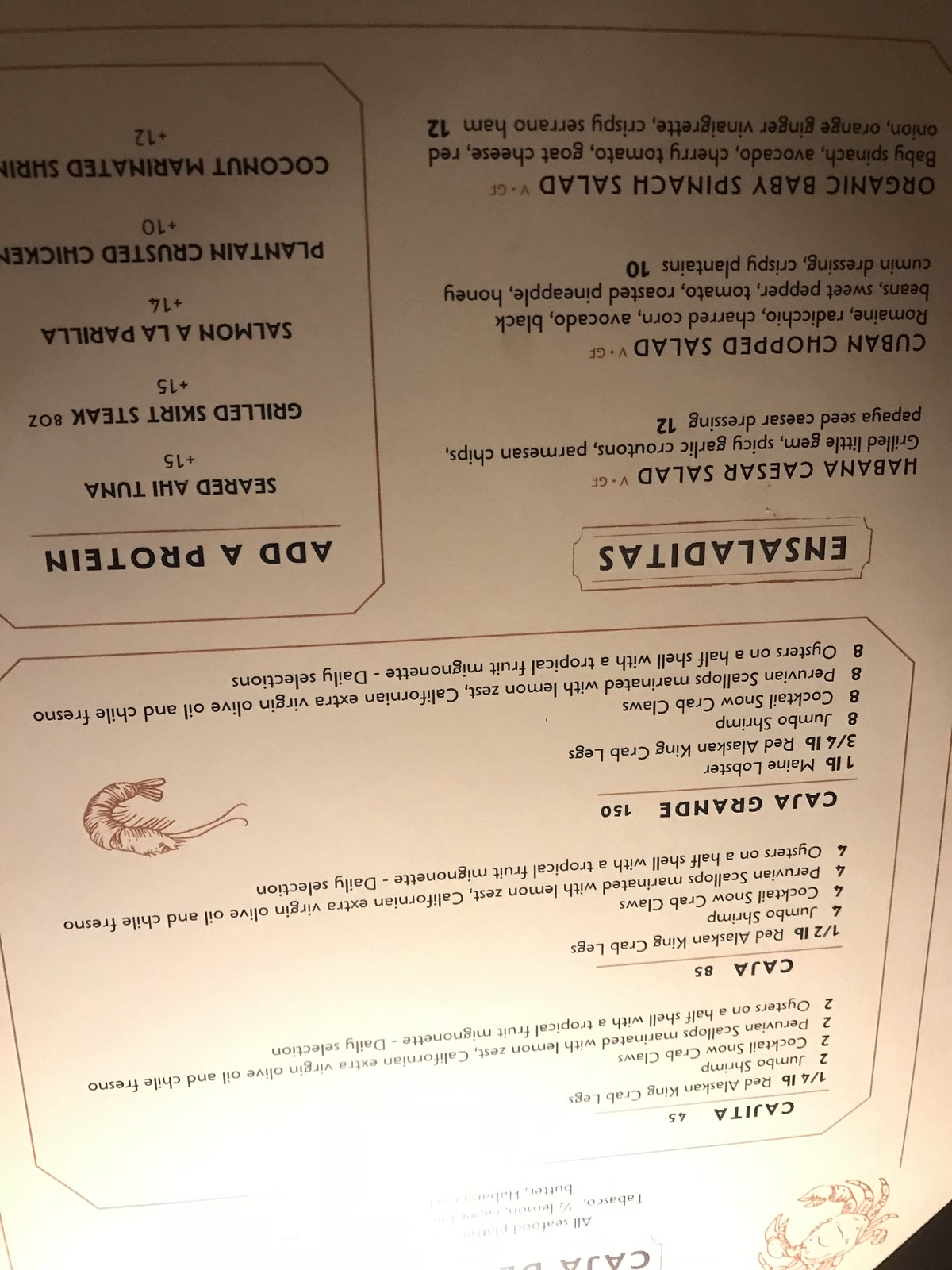In this upside-down photograph, a menu from a seafood restaurant is pictured with intricate details. The primary light source illuminates the menu from above, although it appears at the bottom of the image due to its orientation. The menu itself is either white or cream, embellished with maroon or brown lines. Illustrations of a crab and a shrimp further suggest the seafood theme of the establishment.

The menu's layout includes a section outlined with three dishes, each listed along with their ingredients. Another section, labeled "En Saladitas," likely contains salad options, with additional choices for protein add-ons. All text on the menu is in black, while decorative borders accentuate the headings of various sections, and a thin outline defines each separate section.

The top part of the menu, situated at the bottom of the photograph due to the inversion, is brightly lit, creating a stark white contrast. In contrast, the bottom of the menu (the top of the image) is enveloped in a dark brown hue, possibly due to the lighting conditions.